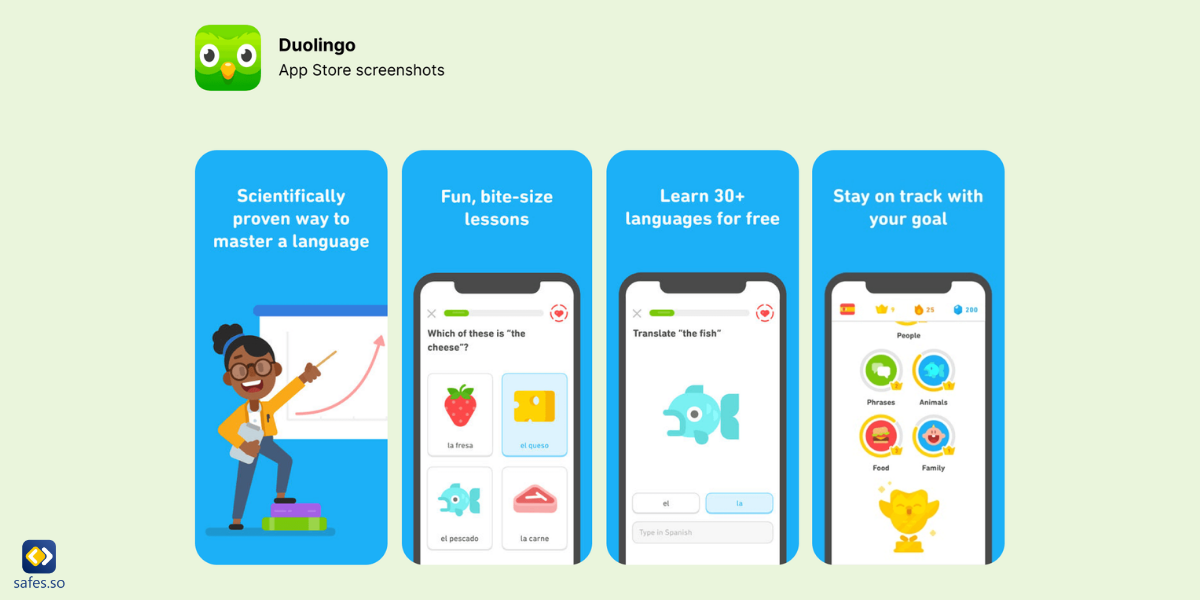This image is a screenshot of the Duolingo app, showcasing promotional content from either the app itself or a related website. Dominating the upper section is the distinctive Duolingo logo—a green square featuring large, white eyes and a yellow beak. Positioned above the icon is the title "Duolingo App Store Screenshots" written in black text against a light green background.

Below the heading are four blue panels arranged horizontally, each containing white text and cartoon-like illustrations:

1. The first panel on the left features an African American female character pointing at a chart. The text reads, "Scientifically Proven Way to Master a Language."

2. The second panel, moving right, shows a smartphone displaying various graphics. The accompanying text says, "Fun Bite Size Lessons."

3. The third panel also has a blue background with a phone illustration showing a fish graphic. The text above reads, "Learn 30+ Languages for Free."

4. The fourth and final panel on the right emphasizes goal-setting. It includes a phone graphic with small icons and an animated avatar, accompanied by the text, "Stay on Track with Your Goal."

These screenshots collectively highlight the key features and benefits of using the Duolingo app.